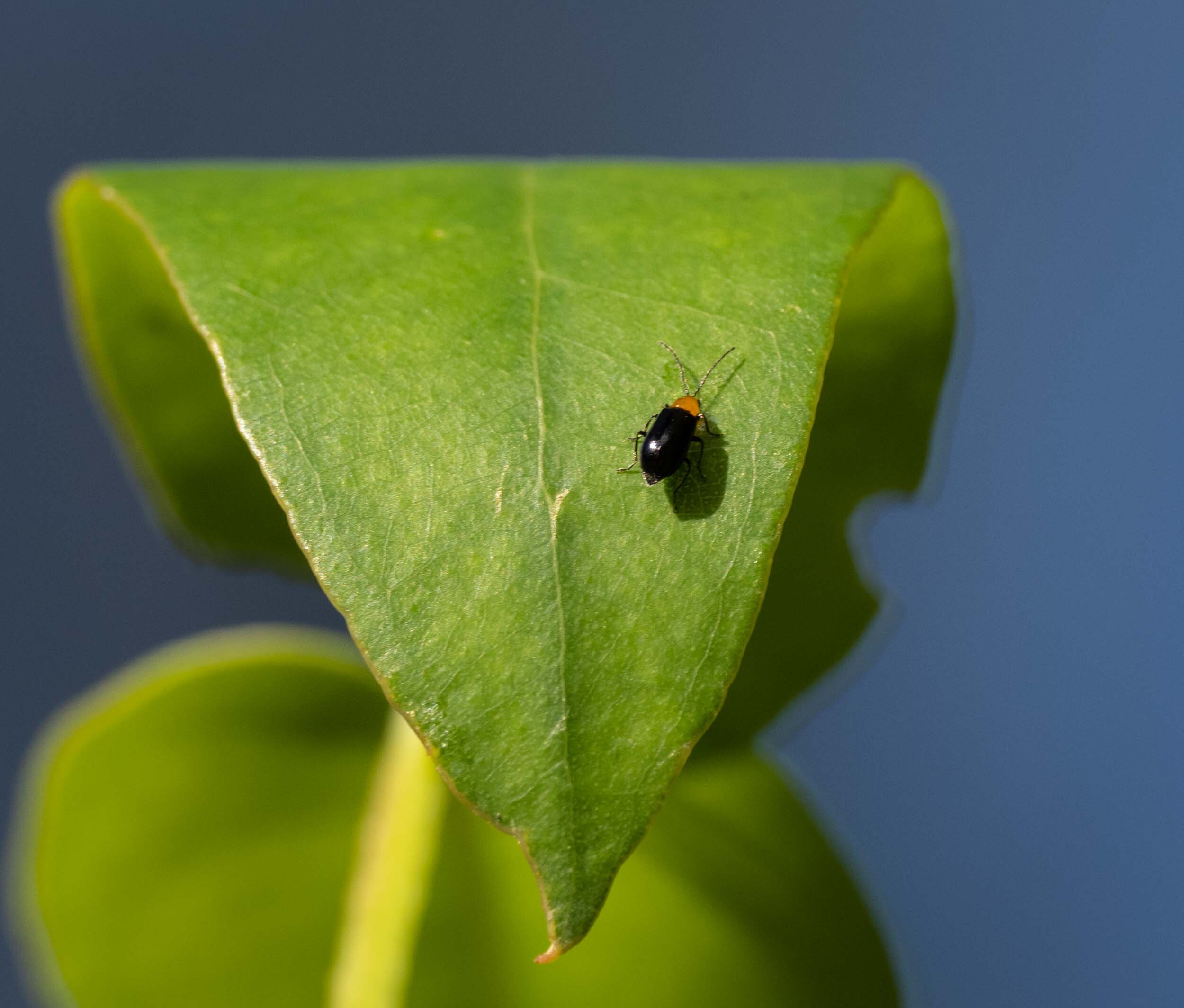In this perfectly square photograph, the focus is on a green leaf that curves downward, forming a triangular V shape with its tip pointed downward. The extreme close-up captures the intricate details of the leaf's surface, which occupies most of the frame and stands out against a background of varying shades of dark blue. The background is somewhat out of focus, enhancing the prominence of the leaf and the subject on it.

Perched on the right side of the leaf, near the center, is a small insect with a black oval body and a striking reddish-orange head. The insect has two antennae and four delicate, thin legs. A vivid shadow of the insect is cast on the leaf by a light source coming from the upper left, suggesting an overhead illumination. The curvature of the leaf and the surrounding shadows add depth to the composition. Slightly blurred leaves and a light green stem can be seen in the background, further emphasizing the main subject in this detailed close-up shot.